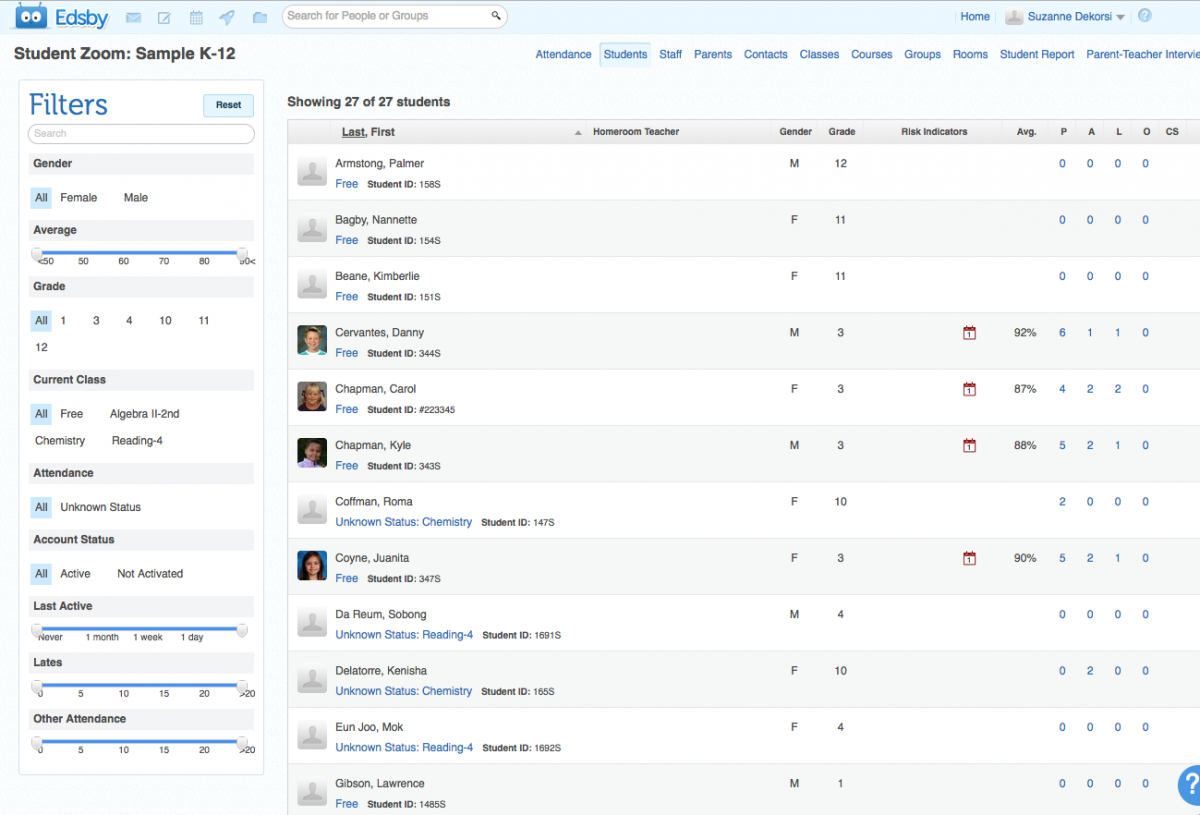Screenshot of the Edsby dashboard on a white background. At the top is a blue rectangle containing the Edsby logo with two small 'I’s. Below the logo is a navigation bar featuring a search bar labeled "Home," followed by the names "Suzanne Davinsky" and "Dekorsi" (spelled D-E-K-O-R-S-I). The navigation links include options for "Students," "Staff," "Parents," "Contacts," "Classes," "Courses," "Groups," "Rooms," "Student Report," "Parent," and "Teacher." The "Students" tab is highlighted in light blue.

The main section of the webpage displays a list titled "Sample K-12 Students," showing 27 of 27 students. Columns in this list include "Last Name," "First Name," "Home," "Teacher," "Gender," "Grade," "Risk Indicators," "Average," and additional abbreviated categories such as "A-B-G-D-O-T-P-A-L-O-C-S." On the left side of the page, there are filtering options with a "Reset" button inside a smaller blue rectangle, situated above another search bar. One column label, presumed to be "Intervention," is truncated to read "I-N-T-E-R-V-I-," highlighting the incomplete display due to limited space.